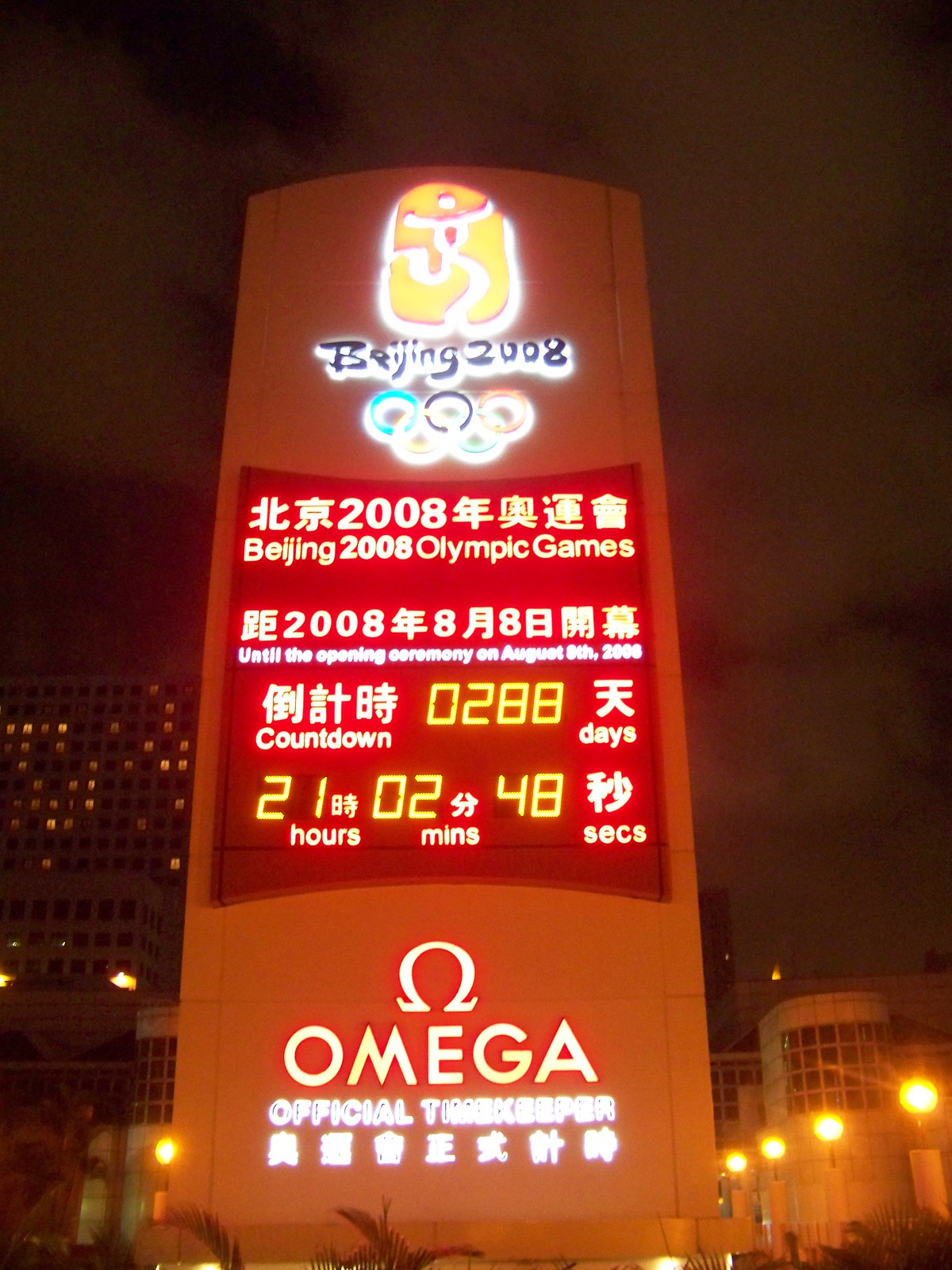The image depicts a large digital display affixed to a massive concrete pillar, set against a nighttime cityscape in Beijing, China. At the pinnacle of the display, a yellow neon symbol illuminates, followed by the text "Beijing 2008" and the interlocked rings of the Olympic logo in blue, yellow, black, green, and red. Beneath the rings, Chinese characters spell out "2008 Beijing 2008 Olympic Games," followed by "Countdown: 288 Days, 21 Hours, 2 Minutes, 48 Seconds." The display indicates that Omega, the official timekeeper for the Games, sponsors the countdown. Surrounding the display is the illuminated city, with large office buildings visible in the background. The night sky appears cloudy, adding to the diffuse glow of the city lights.